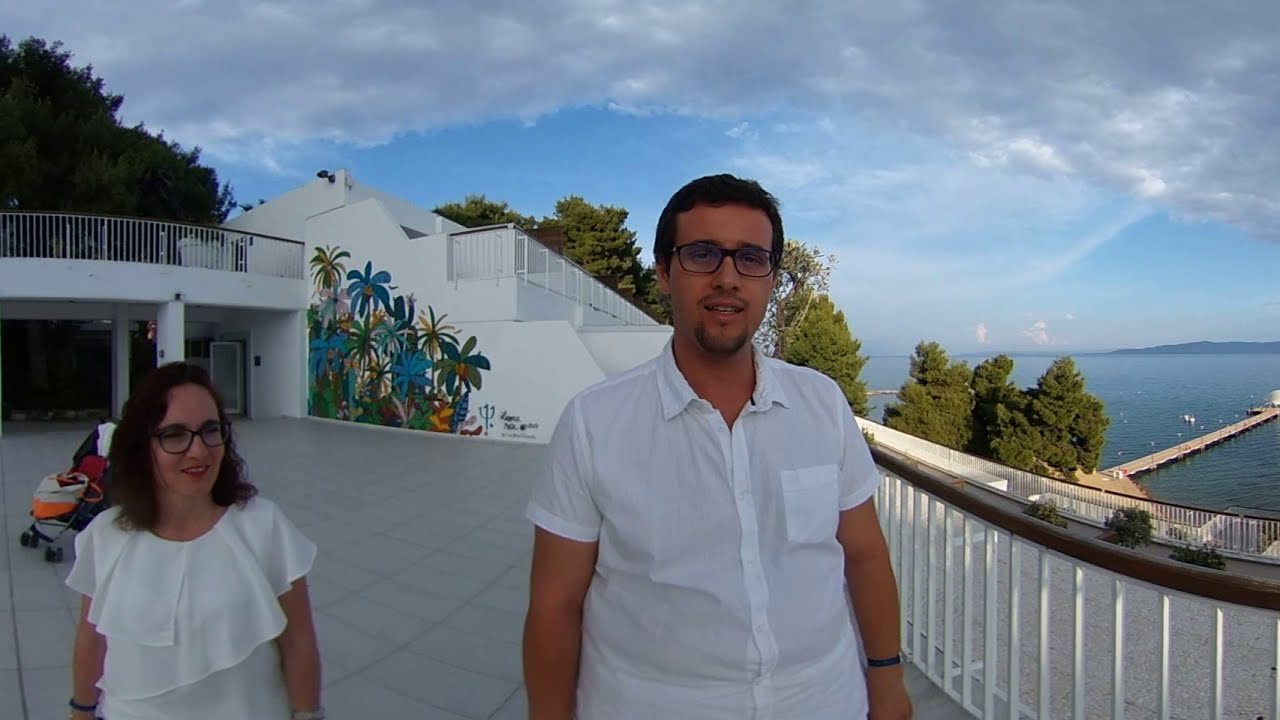A man and a woman stand together in a scenic setting that combines seaside charm with artistic architecture. The man, who occupies the center of the frame, is wearing a white button-up shirt with a pocket and glasses. His short black hair and goatee give him a distinguished look. The woman, positioned to the bottom left corner of the image, has medium-length brown hair and also wears glasses. She is dressed in a white blouse and has a black band on her wrist, similar to the man. She stands beside a baby stroller draped in an orange and beige bag.

In the background, a multi-level white building adorned with a vibrant mural of palm trees and other plants adds a splash of color and life to the scene. Adjacent to the building, a guardrail lines a raised walkway, hinting at a complex architecture that includes a door, balcony, staircase, and terrace. 

On the right side of the image, a dock extends out into a vast body of water that reflects the blue sky peppered with grey and white clouds. The scene is framed by a lush array of trees, enhancing the picturesque quality of the setting. The paving beneath them is grey tiled, indicating a well-maintained area suited for leisurely strolls. The overall impression is one of harmony between the built and natural environments, under a bright daytime sky.